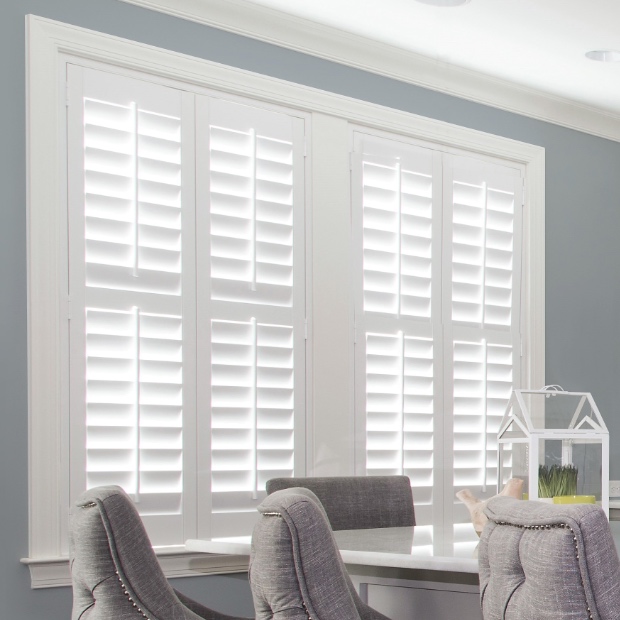The photo captures a serene and elegant interior of a home, highlighting a cozy and stylish dining area. Dominating the scene is a large window framed in white, featuring horizontal shutters that are predominantly closed, allowing only slivers of light to filter through. The wall surrounding the window is painted a soft gray, contrasting with the white molding that crowns the gray walls and matches the white ceiling. In the foreground, a white-topped table with a solid gray base is partially visible. Surrounding the table are several upholstered chairs, adorned with light and dark gray striped fabric and accented by silver metal studs, adding a touch of sophistication to the setting. On the table, a chic decorative piece—a white greenhouse with glass sides housing a vibrant green plant—catches the eye. Nearby, a light pink ceramic bird adds a whimsical touch to the arrangement, contributing to the overall charm and warmth of the space.